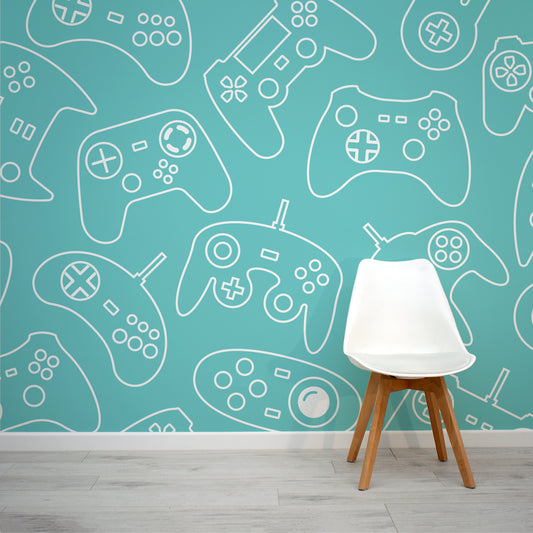The image showcases a modern room with a light gray laminate floor that spans the entire frame. Positioned in the bottom right corner is a sleek white plastic chair with curvy lines and no armrests, supported by four light brown wooden legs. The wall behind the chair is adorned with a playful, kid-themed wallpaper in a seafoam green or teal color, featuring detailed white outlines of various video game controllers. These controllers include recognizable designs such as those from the Super Nintendo, Xbox 360, PlayStation 4, Sega Genesis, and Nintendo 64. Scattered across the background, the controllers vary in shape, with some being more curvy or pointy, each adding to the lively and nostalgic decor of the room.